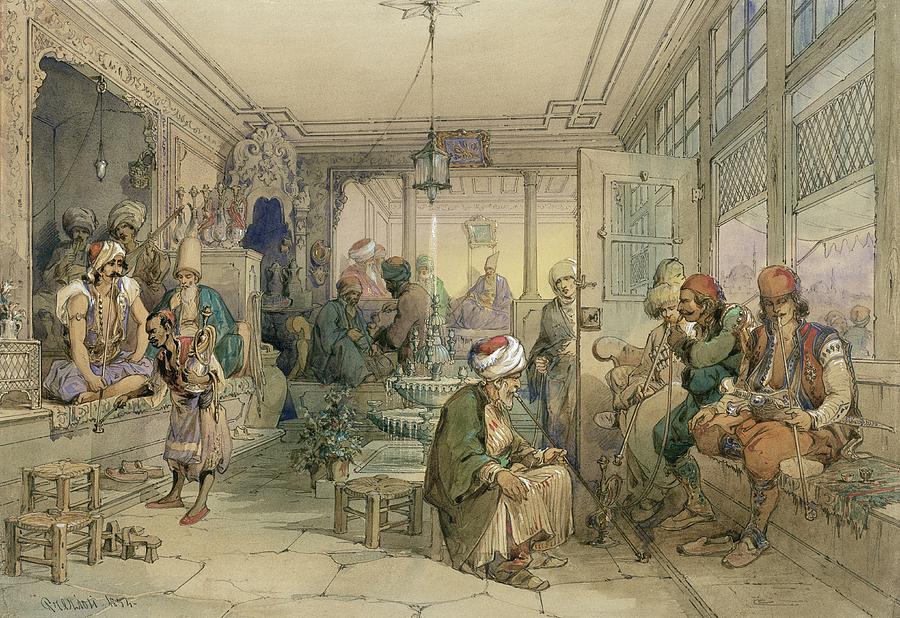The illustration portrays a bustling scene set in a historical Middle Eastern room, possibly from the 17th century. The artwork is not photorealistic but rather has a drawn, book-illustration quality to it. Inside the room, various men are gathered, dressed in an array of traditional Middle Eastern attire that includes long robes, sashes, turbans, vests, and moccasins in hues of green, blue, and red. The men are seated on benches along the room's sides and on stools positioned centrally, engaging in conversation and smoking long pipes, indicating a hookah lounge setting. A small, ornate two-layer fountain is the centerpiece of the room, with water gracefully arching into the air. The decor suggests an old-style, almost Victorian atmosphere with intricate architecture and a central hanging light fixture. Additionally, a person is seen serving hookah to the seated groups, enhancing the lively yet historical ambiance of the scene.